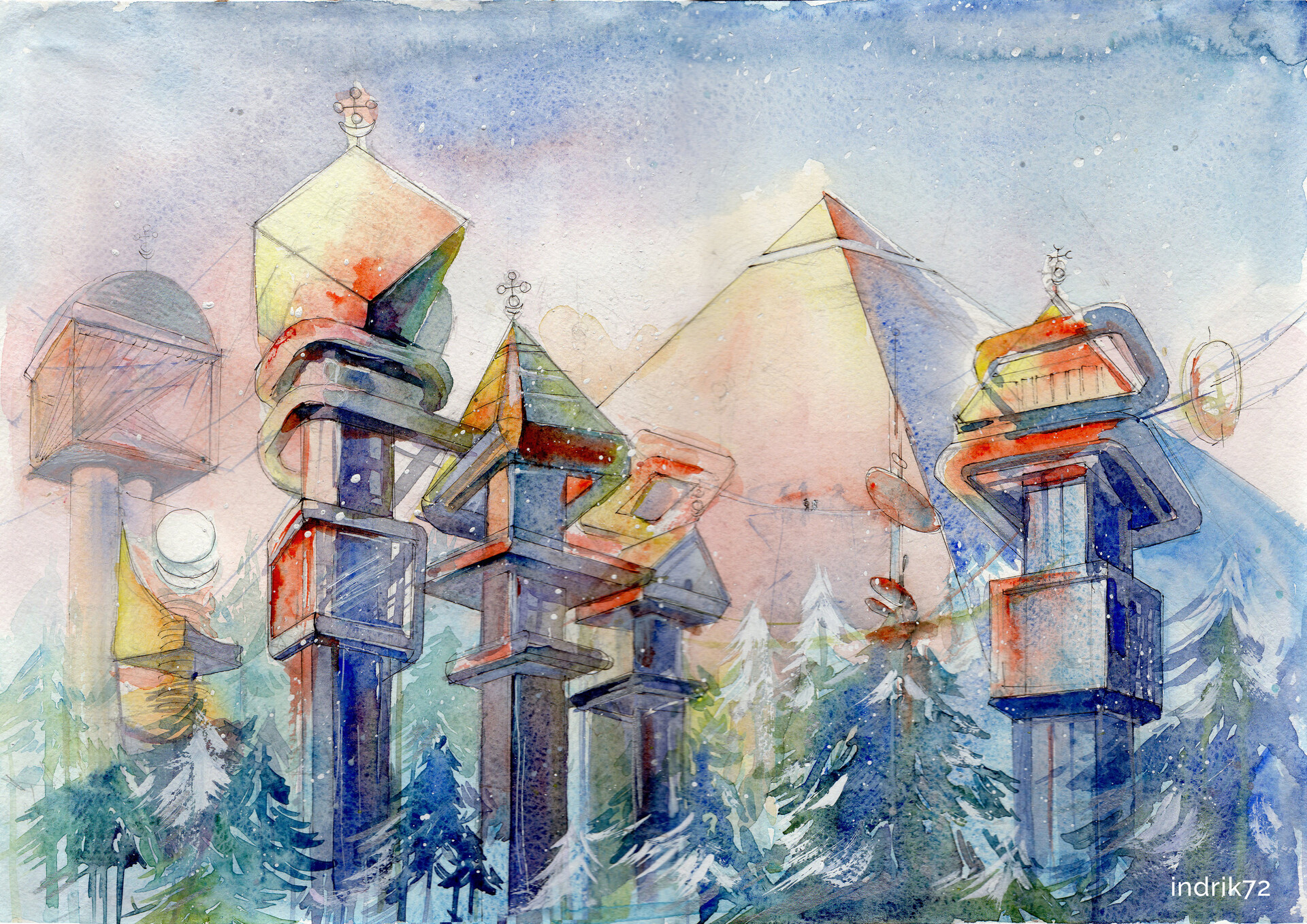In this watercolor painting, a futuristic landscape is depicted with striking detail and vibrant colors. Dominating the background is a grand pyramid with its top section distinctly separate from the rest of the structure. In front of this pyramid, five long, rectangular towers stand tall, with four positioned on the left and one on the right. The towers vary in color, featuring a transition from dark blue to light blue on the right side, and from light yellow to orange on the left side. Some of these towers have cube or pyramid shapes at their tops, adorned with what appear to be rotating square links, adding a sense of movement and alien-like technology. The scene is populated with green pine trees dusted with white snow, enhancing the otherworldly ambiance. In the sky to the right of the pyramid, a celestial body resembling the Sun or the Moon glows softly. The entire composition is brought to life with a palette of blues, greens, tans, yellows, reds, grays, and off-whites. The bottom right corner of the painting is signed with the name "INDRIK72," likely the artist's signature, adding a final touch to this unique and surreal watercolor.